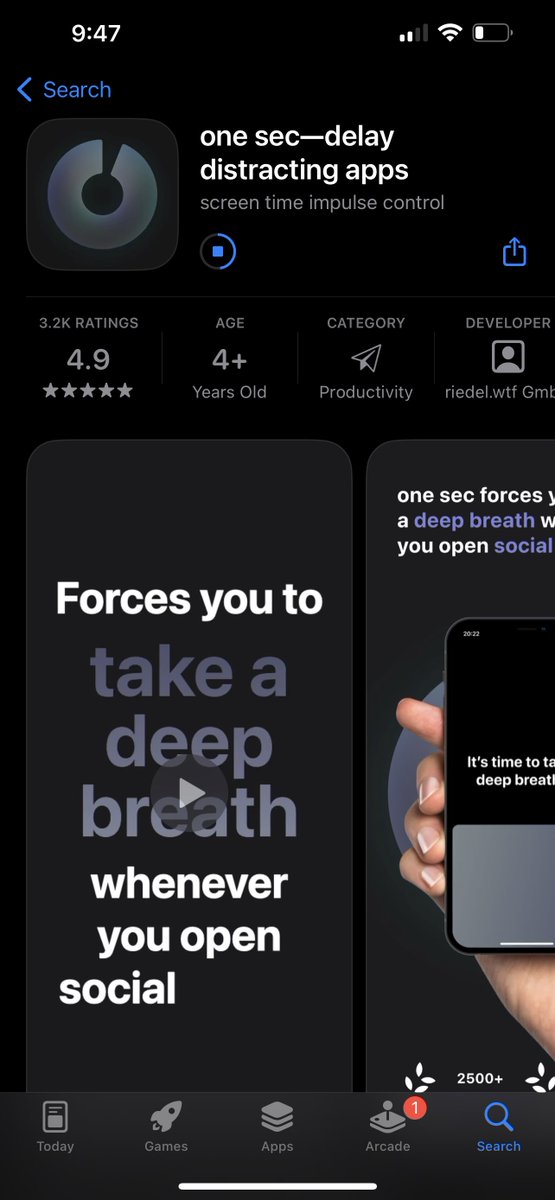The image depicts a screenshot from a tablet or smartphone, identifiable by the icons and symbols located in the top-left corner, including the time (9:47), Wi-Fi signal strength, and wireless service indicators. The device's battery icon is nearly depleted. Below these icons, a blue search bar features a back button, indicating the user is navigating within an app store.

The screen displays the details of an application named "OneSec Delay Distracting Apps: Screen Time Impulse Control," which appears to help users manage their time on distracting apps by introducing a delay. The app boasts 3.2 thousand ratings and a stellar average rating of 4.9 stars. It is suitable for users aged 4 and older and falls under the Productivity category. The developer is identified as RIDAL.WTF.

Beneath the app’s name, a description indicates that OneSec forces users to take a deep breath before accessing social media apps. An accompanying image includes a play button and shows a person holding a button, reinforcing the app's functionality. The bottom of the screen showcases the navigation bar with tabs labeled "Today," "Games," "Apps," "Arcade," and "Search." The white home bar, typical of modern Apple devices, is also visible.

Overall, the screenshot captures an app store interface promoting a productivity app designed to manage screen time and reduce impulsive access to distracting applications.